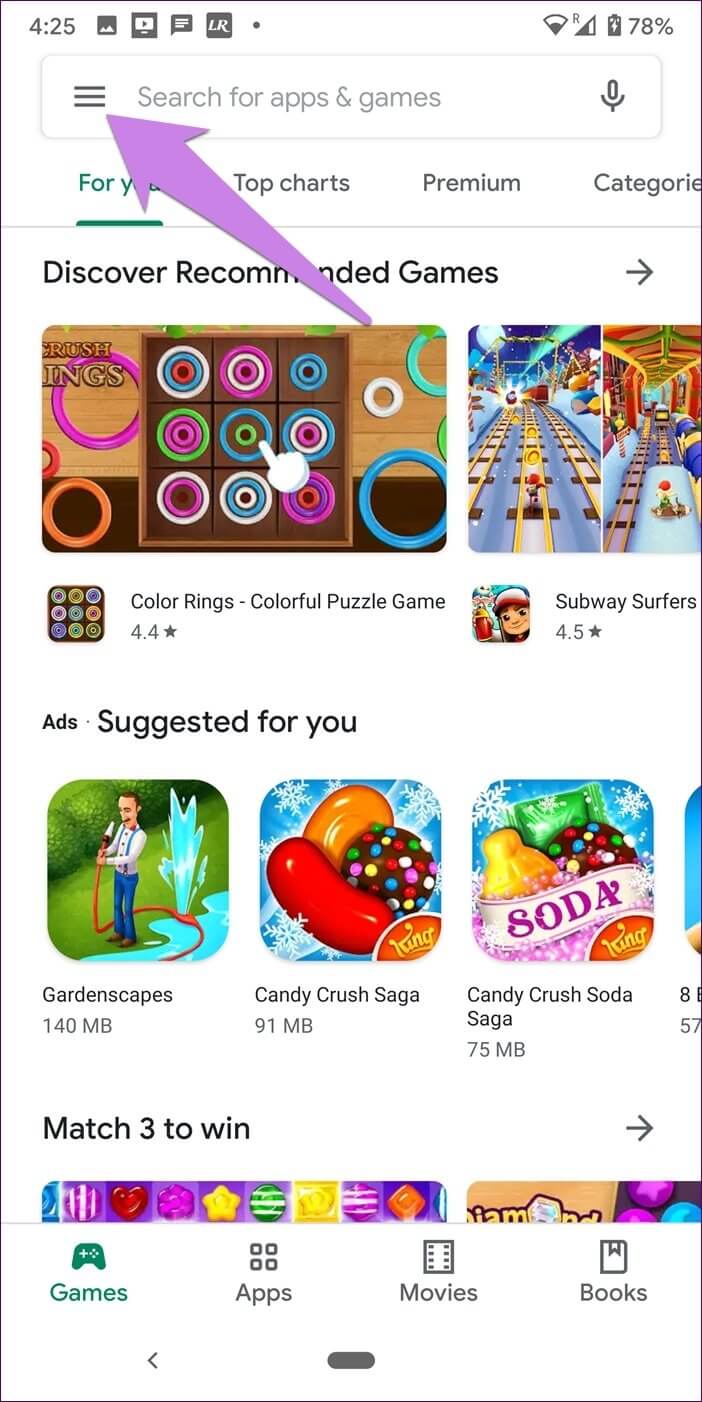The image is a vertically rectangular screenshot from Google Play, featuring a predominantly white background at the top. At the very top, the time is displayed as 4:25 PM in dark gray text. Multiple icons indicate various notifications, including a text notification and a screenshot or image save notification. On the right corner, the Wi-Fi signal bar, battery icon, and battery percentage (78%) are visible.

Just below this top bar, a large search field labeled "Search for apps and games" is prominently displayed. Overlaying the image is a large purple arrow, originating from about a third of the way down the image and pointing upward towards the three horizontal bars icon located on the right side of the search field.

Below the search field, several tabs labeled "You," "Top Charts," "Premium," and "Categories" are visible. Beneath these headers, the section "Discover Recommended Games" showcases a few featured games such as "Color Rings," "Colorful Puzzle Game," and "Subway Surfers."

Further down, the section "Ads Suggested for You" highlights popular games like "Gardenscapes," "Candy Crush Saga," and "Candy Crush Soda Saga." Despite part of the next section, "Match 3 to Win," being cut off, it indicates more recommended games that would require scrolling to reveal in full.

At the bottom of the screenshot, the navigation options include "Games," "Apps," "Movies," and "Books."